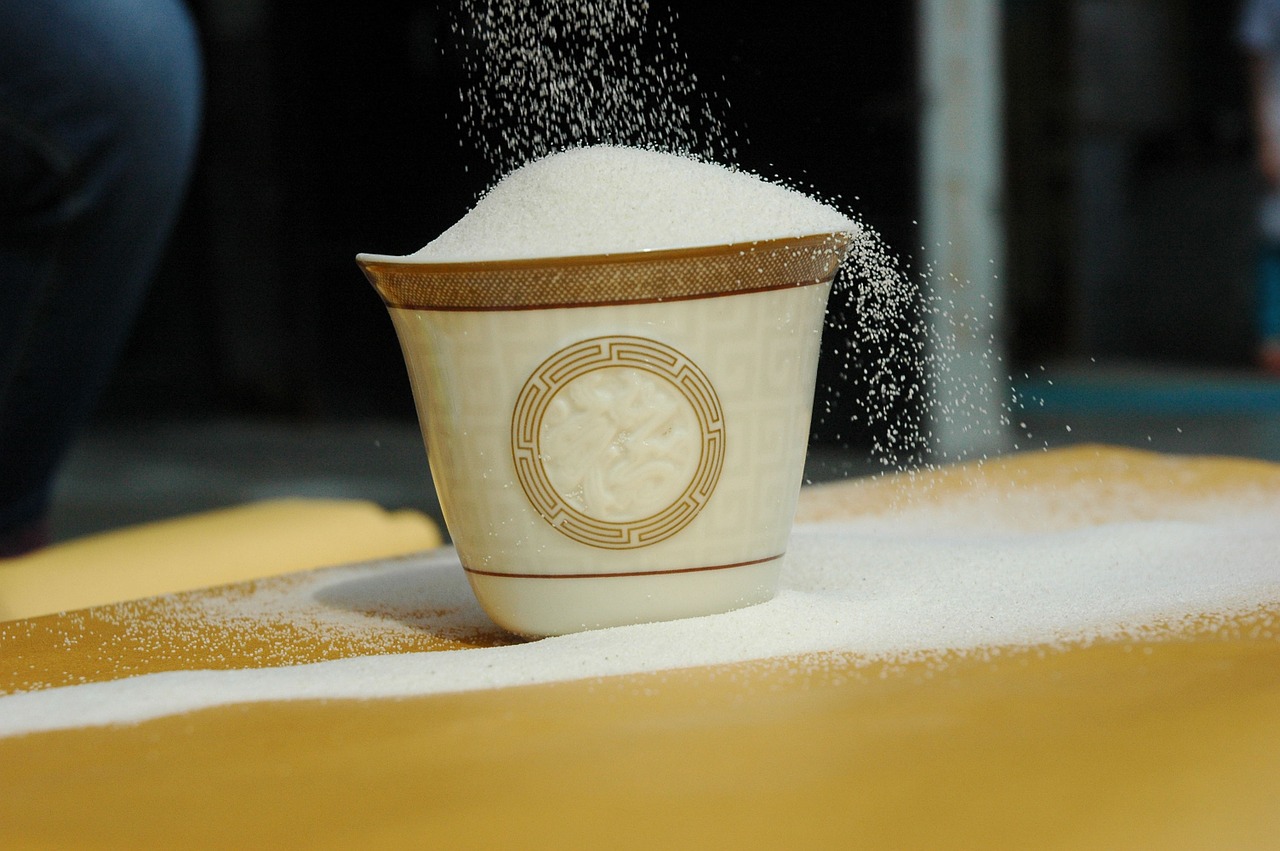The image depicts a beige and brown ceramic mug placed on a yellow table, overflowing with fine white granulated crystals, likely salt. The mug, which features a circular maze design in the center, is being filled from above, causing an abundant spillage that forms a heap of white crystals on the surface below. In the background, there is a blurred, bluish-grey interior setting, and part of a person’s leg dressed in what appears to be dark blue jeans is visible on the left side.